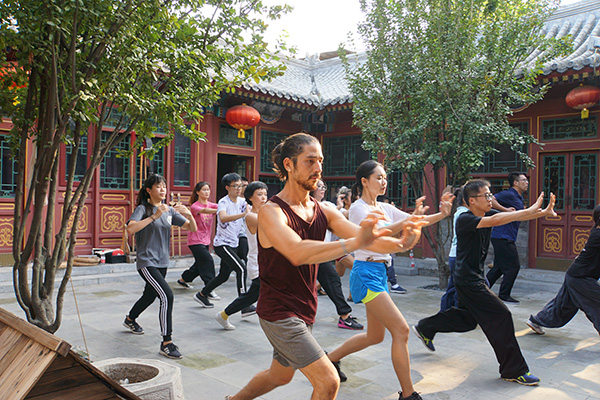The image captures a color photograph in landscape orientation, showcasing a group of about 15 people engaged in a Tai Chi session in the courtyard of a Buddhist temple complex. The courtyard features a gray cement floor and is adorned with oriental decorations, such as hanging red lanterns and a few small green trees in pots, possibly crepe myrtles. In the background, a one-story red building with a low pagoda-style roof and golden accents can be seen, enhancing the traditional Asian aesthetic of the scene.

The participants, primarily of Asian descent with one Anglo man sporting a ponytail in the foreground, are spread across three visible rows. They are all facing the bottom right corner of the image, uniformly lunging forward on their right legs with their left legs extended behind them. Their arms are outstretched in front of them, many with bent elbows and claw-like hand positions. The group is dressed casually in a mix of workout attire, ranging from long tracksuit pants to shorts. Notably, one woman stands out in bright turquoise shorts with yellow lining, while the rest of the clothing palette consists of subdued blacks, grays, and browns. Despite the absence of a visible instructor, it appears that everyone is focused ahead, possibly following unison Tai Chi movements.